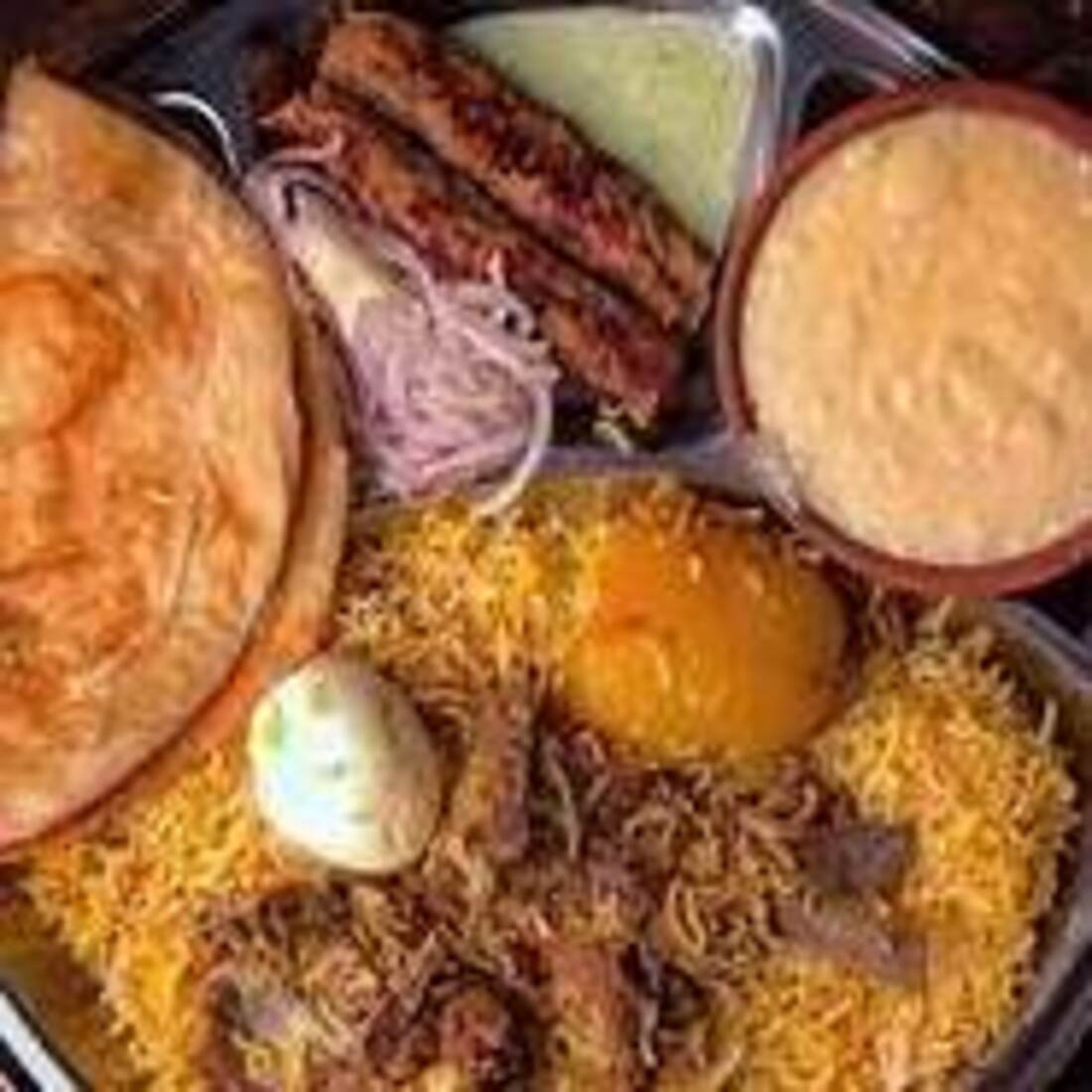This close-up, slightly blurry image showcases a seemingly foreign breakfast spread, which may be unfamiliar to viewers from the United States. Central to the meal are sausage links situated at the top alongside what appears to be shredded onions. To the left, there are round, flat items that seem to be either pancakes or corn cakes. Below this, there is a single hard-boiled egg perched atop a bed of shredded food, possibly mixed with meat. Additionally, a yellowish substance, resembling fried rice, is visible, adding a colorful element to the dish. Towards the top-right, there's a red dish containing a substance that might be beans or grits. A green sauce can be seen beneath what looks like enchiladas, which are located above the rice. Lastly, a batch of tortillas and a dollop of sour cream complete the meal, further hinting at a do-it-yourself breakfast burrito kit. Despite the blurriness, the array of elements suggests a rich and diverse breakfast plate.